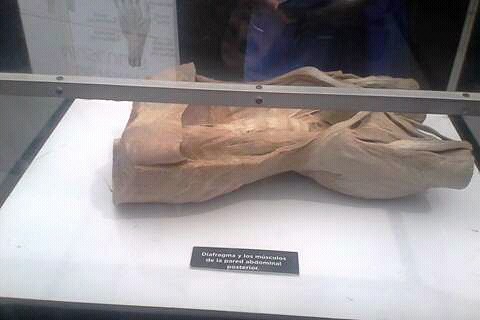This image depicts a museum artifact showcased within a glass case. The artifact appears to be a large piece of wood or driftwood with a rich color gradient, transitioning between muted brown and a reddish-brown hue. The wooden piece, intricately hollowed out in some areas, spans almost the entire width of the case and exhibits a rectangular and horizontal orientation.

The glass case is held together by a metal frame, visible at the top of the image, with silver bars and darker gray knobs securing the structure. A prominent feature of this display is a small black tag placed on the white surface at the bottom of the case. The tag contains white text, likely in Spanish, although the exact inscription is indiscernible.

Also noticeable in the background is a diagram, suggesting that the setting is indeed a museum. Additionally, there seems to be a reflection or shadow of a person on the glass, indicating that the viewer is standing close to the exhibit, further emphasizing the context of this being an artifact on display.